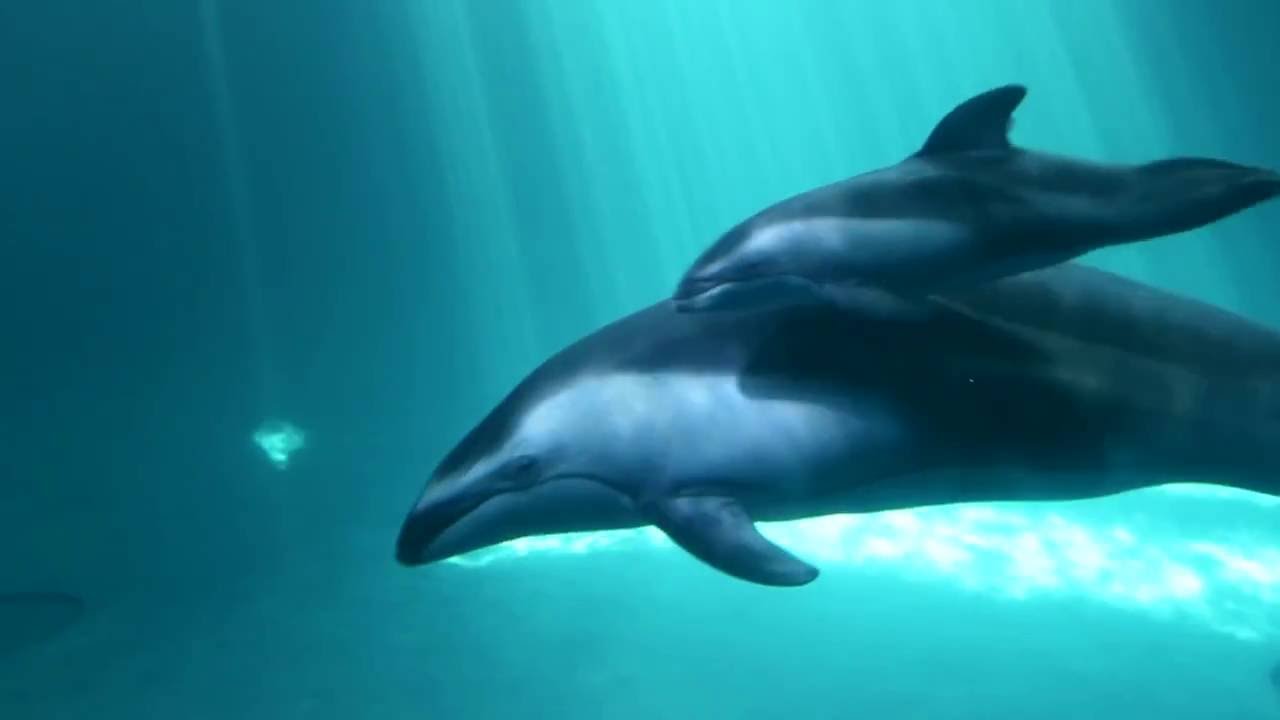This is a realistic image featuring two dolphins swimming underwater in what appears to be a tranquil ocean. The scene, set in a rectangular frame wider than it is tall, captures a mother dolphin and her baby gliding through turquoise waters from right to left. The dolphins are a dark gray color with lighter underbellies, and they display a distinctive curved, frowny mouth. The mother dolphin, about three feet long, has a fin visible atop her body, and her baby, approximately one to two feet in length, swims just above her, casting a shadow onto her back. Surrounding the dolphins, rays of sunlight pierce through the water from the surface, creating white streaks that illuminate the scene. At the bottom left of the image, there's a mysterious glowing blue object, possibly a jellyfish or a play of light reflection. The overall ambiance is serene, with the vibrant blue and sea green hues of the ocean contrasting beautifully with the dolphins' sleek gray bodies.